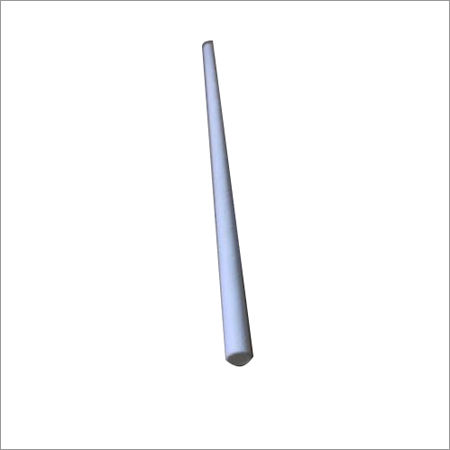The image depicts a stark, minimalistic scene with a vertical rectangular box set against a white background. Central to the image is a cylindrical rod, subtly skewed to the left and extending vertically. The rod, primarily a blend of bluish, silverish, and white hues, appears metallic or plastic and projects a three-dimensional quality that makes it seem longer and extending into the distance. It has smooth, seamless surfaces and a slight black trim with a definite black bottom, possibly to enhance a shadow effect and accentuate its form. It appears hollow or could have an object at one end, though this detail is not entirely clear. The rod, resembling a dowel but in more futuristic colors, occupies the central focus of the image, suggesting it is intended to be showcased.